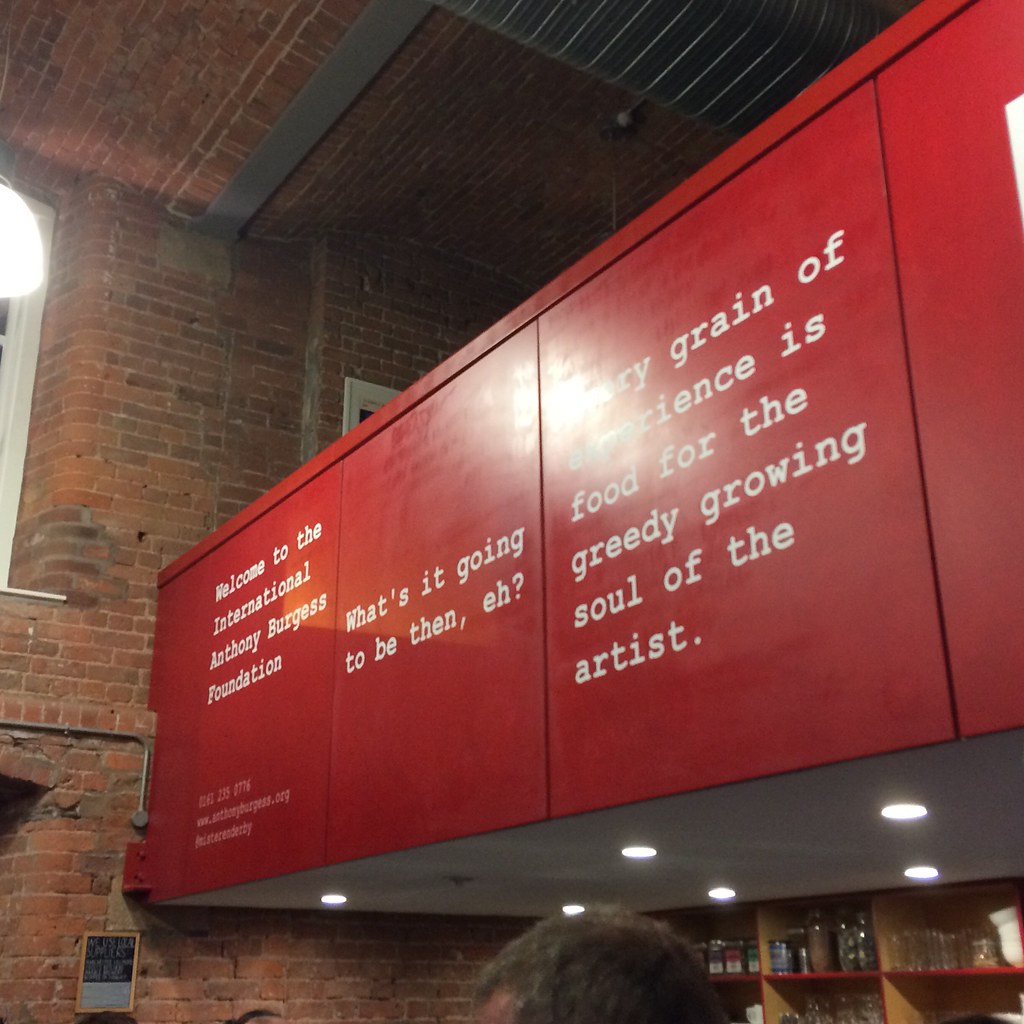In a cavernous, repurposed industrial building with exposed brick walls and a ceiling, a prominent red sign catches the eye. This sign, written in white text in Courier font, reads "Welcome to the International Anthony Burgess Foundation," paying homage to the author of "A Clockwork Orange." The sign is mounted on the outer wall of a balcony, which also serves as a light source with embedded lighting. Below the sign, a smaller, partly obscured quote states, "Every grain of experience is food for the greedy growing soul of the artist." The room, possibly a coffee shop or gathering place, has a cozy ambiance with shelves lined with jars, bottles, and glasses, hinting at food service or artistic activities. Windows with white trims add to the visual symmetry. The partial view of a man's head at the bottom of the image suggests he might be waiting in line, adding a human touch to the bustling scene.